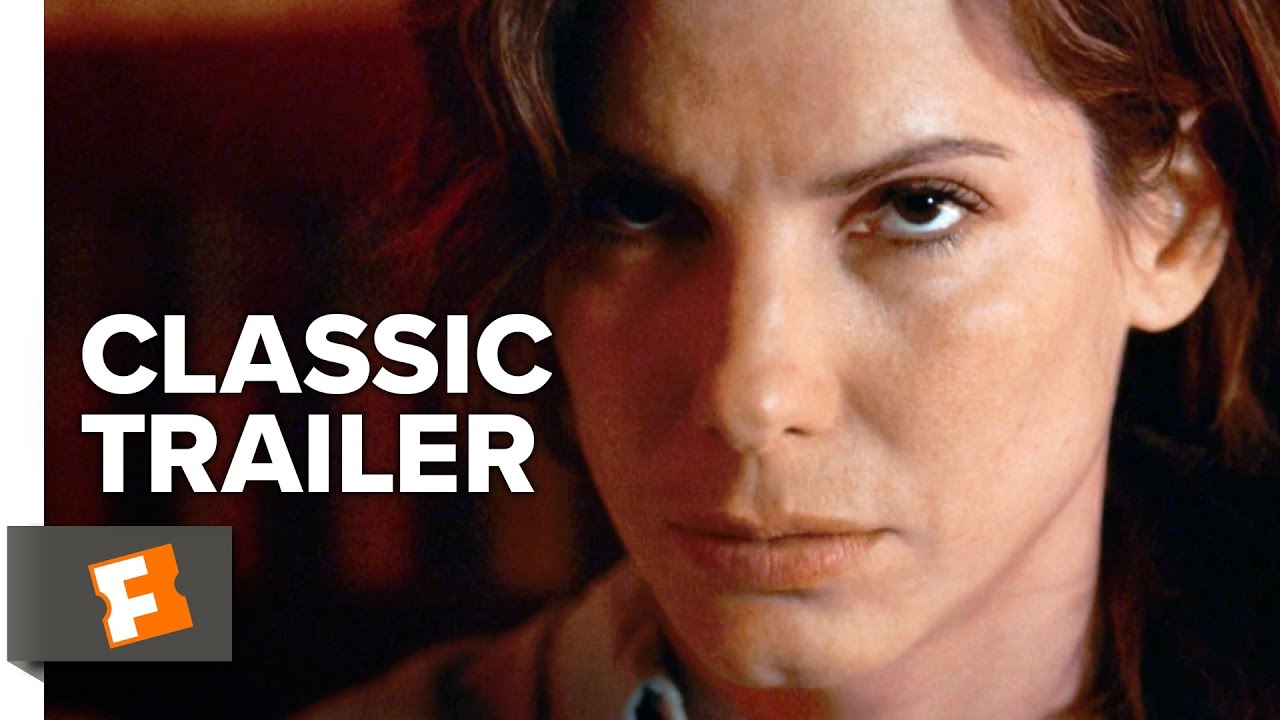This is a close-up, horizontally aligned rectangular image with no border, capturing the stern face of a slightly younger Sandra Bullock. The focus is solely on her face and a bit of her neck, with her head facing directly towards us while her eyes glance upward, giving her an angry or upset expression. Sandra, a Caucasian woman, has brown hair framing her face and extending longer behind her ears. The background on the left side is blurred with medium to dark brown colors. Centered on the left in all-capital white sans-serif text, the words "CLASSIC TRAILER" are stacked one above the other. Below the text, there's a logo featuring a white capital 'F' on an orange ticket stub, placed against a gray rectangular background, signifying Fandango.